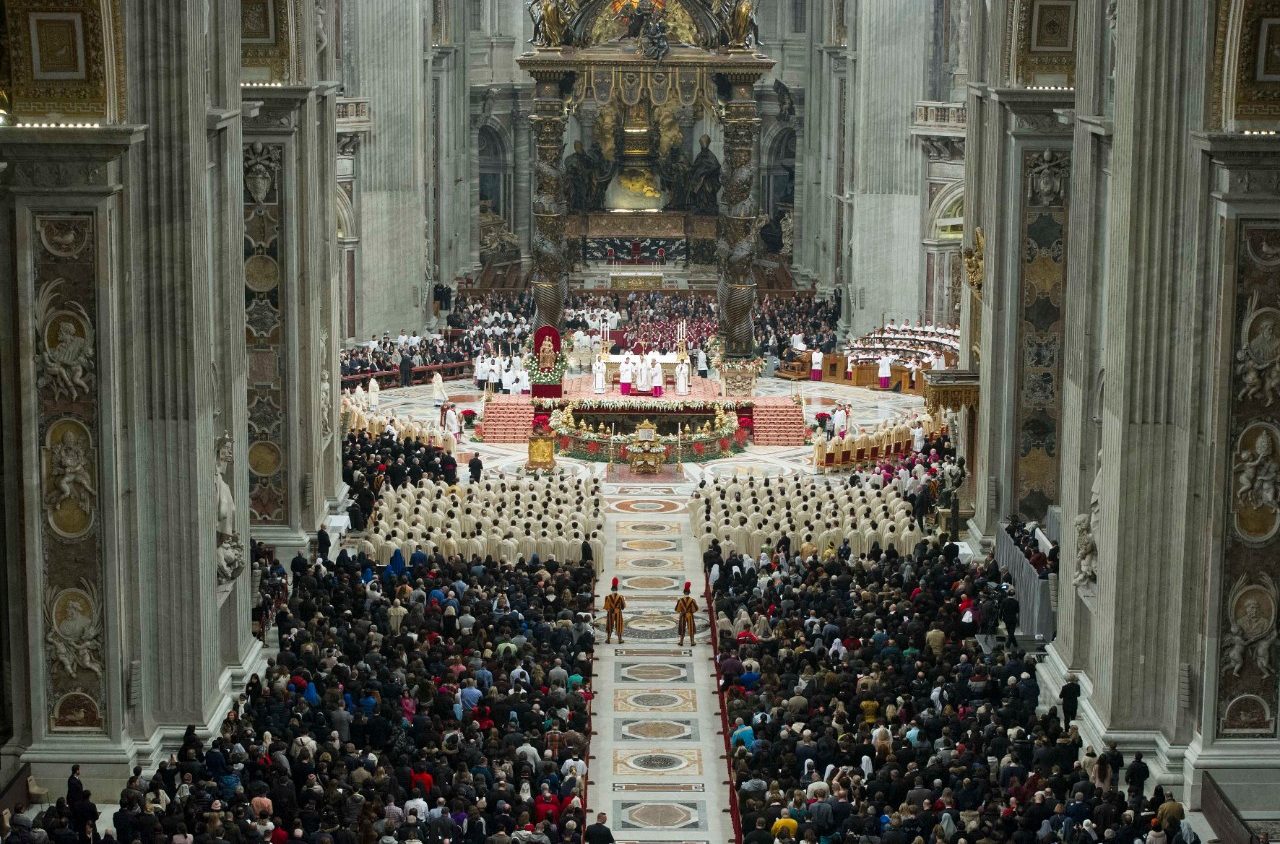The image is a large, detailed color photograph depicting the grand interior of a cathedral, likely the Vatican, during a significant church service, possibly on Easter or Christmas. Towering gray pillars line the sides of the cathedral, leading the eye to a central corridor filled with congregants. The focus appears to be on the central aisle, which is flanked by groups of people. In particular, many individuals are adorned in white clerical robes, some accented with pink, suggesting their official roles in the ceremony. Toward the front, two figures stand out in their colorful outfits of yellow, red, and blue. Regularly dressed people fill the background, adding to the sense of a densely packed, majestic space. This image captures the solemnity and grandeur of the occasion, hinting at the presence of a high-ranking religious figure, perhaps the Pope, although the image composition makes it difficult to discern any specific individual at the altar.